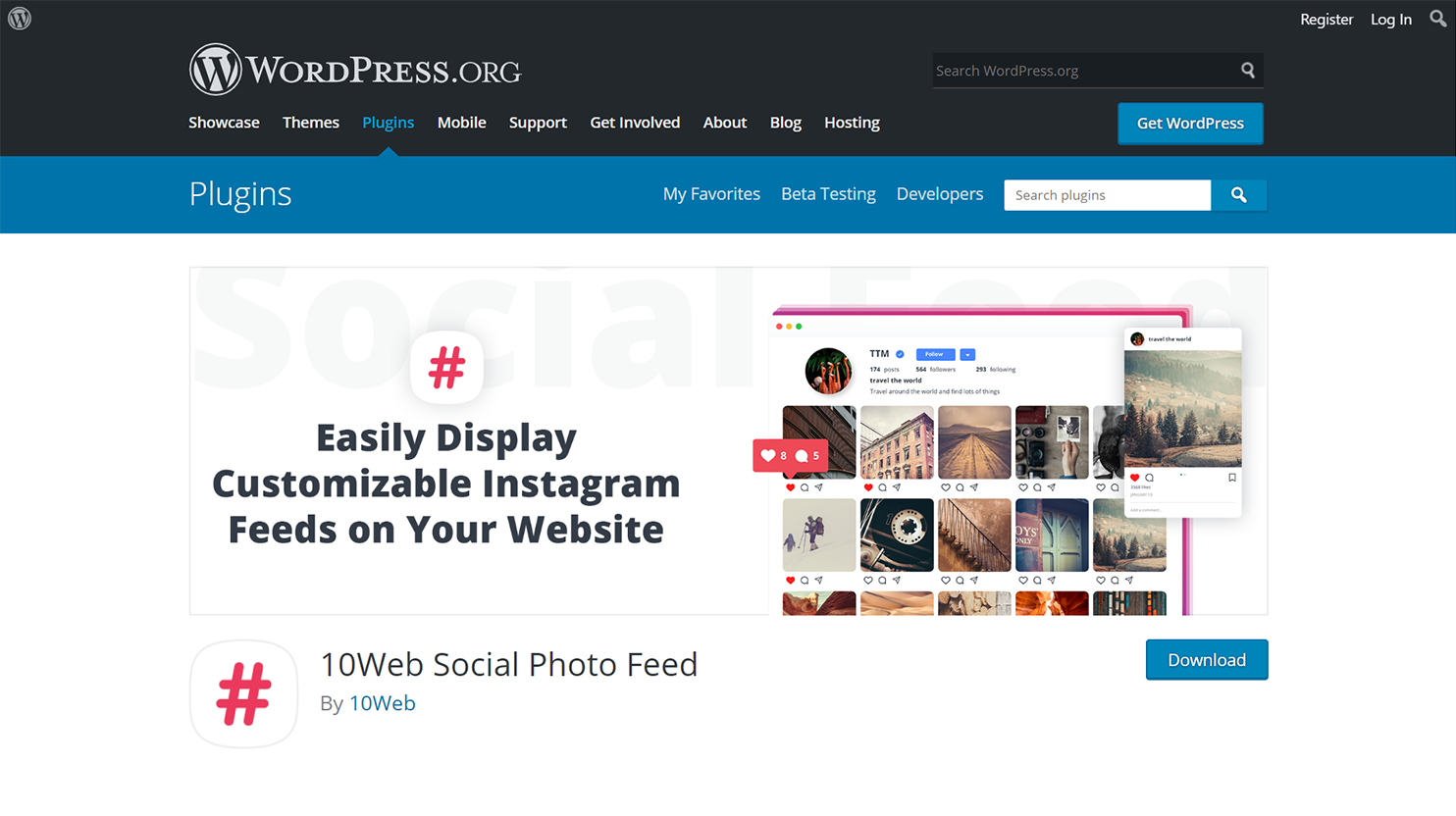Here is a cleaned-up and detailed caption for the image:

---

This screenshot features the "Plugins" section of the WordPress.org website. At the top left, the header displays the word "Plugins," while the top right section includes options such as "My Favorites," "Beta Testing," and "Developers." A search bar positioned to the far right has the placeholder text "Search plugins" in small gray letters. Beneath the blue header line, the website background is predominantly white.

On the right side of the screen, there is a preview image of an Instagram page, showing a feed filled with thumbnails. The top right corner of this preview page features icons for liking and commenting, along with a smaller overlay of the Instagram user's feed. The bottom right section of this preview displays a "Download" button. Adjacent to this button, the text "Hashtag 10Web Social Feed by 10Web" is shown, identifying the plugin.

---